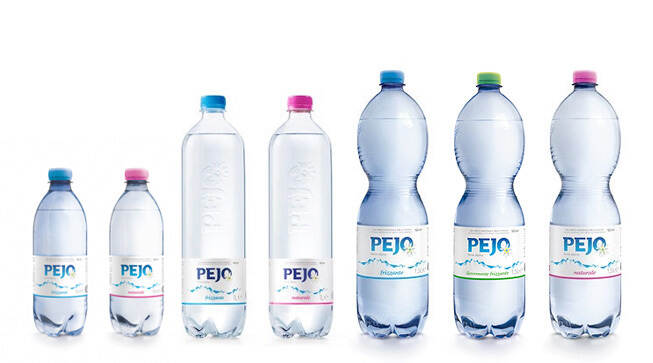A series of seven water bottles from the Pejo brand are arranged from left to right, showcasing different sizes and colors. On the left, there are two smaller bottles with white labels featuring the brand name "Pejo" in blue text and a star at the bottom of the "O." These bottles, which are about 16 ounces or a half-liter each, have matching blue and pink caps and corresponding color borders on the labels. In the middle, two taller, round bottles have blue and pink caps with matching color lines on their labels. On the right, three larger, curvier bottles are approximately a liter or taller, each with a blue, green, or pink cap, again with matching color borders on the labels. All bottles are made of plastic and are filled with water, suggesting that the different cap colors might indicate various flavors or types of water.